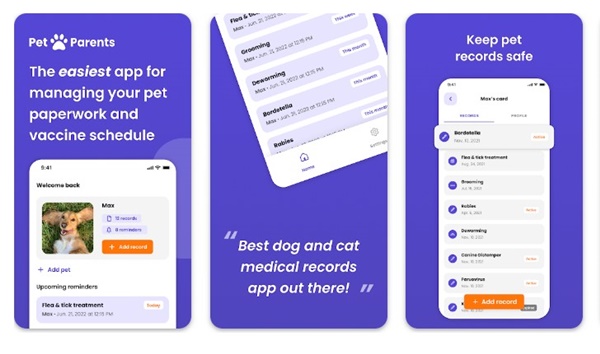In this image, we see three neatly organized stacks of cards, each adorned with unique design logos. The topmost card stack features text that reads, "Pet Parents: The easiest app for managing your pet paperwork and ration schedule. Welcome back, Max. Upcoming reminders: flea and tick treatments." The middle stack of cards includes references to "grooming, daydreaming, and vaccines," while the lower stack indicates "rabies vaccinations" and mentions the "best dog and cat medical records app" for keeping pet records safe. There is also a card for Max with reminders for "flea and tick treatments, grooming, and rabies vaccinations." The image is predominantly colored in shades of orange, blue, white, and brown, offering a visually appealing and organized display of pet care management tools.